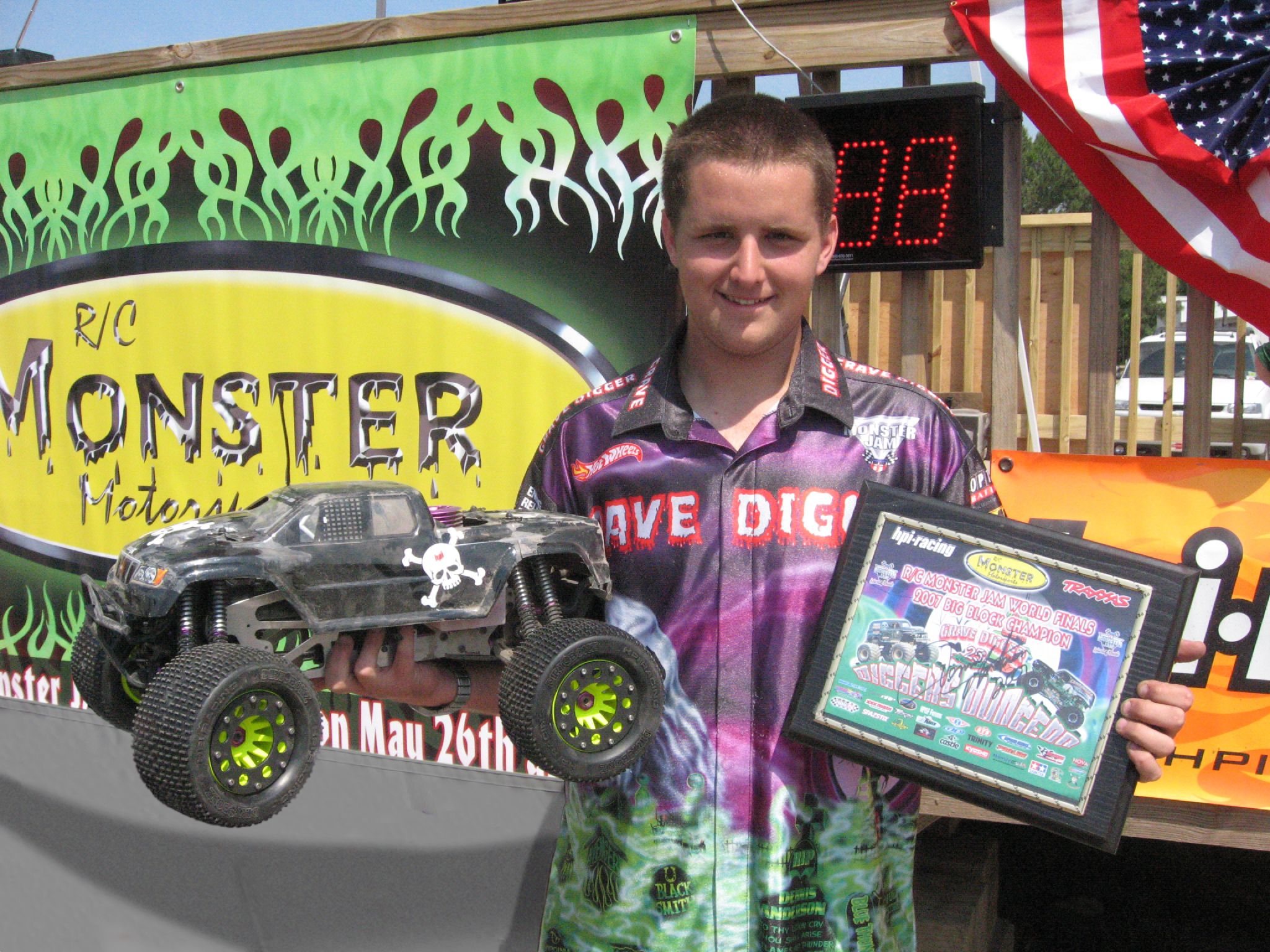In this outdoor image, a young white male with short brown hair is positioned towards the right-hand side, prominently smiling and squinting at the camera. He wears a vibrant and multicolored shirt that is black, purple at the top, and green at the bottom, featuring a 'Gravedigger' logo with a red border and a Hot Wheels logo. In his right hand, he holds a black toy monster truck with four large wheels. His left hand carries a framed certificate that reads "RC Monster Jam World Finals 2007 Big Block Champion," adorned with pictures of monster trucks and various advertisements. Behind him, visible elements include a backdrop bearing the text "RC Monster Motor," parts of a wooden deck area, and in the upper right corner, an American flag with red and white stripes and a blue field of white stars. There's also a digital sign displaying '88' and a green sign with a yellow and black oval, partly obscured. A notable element in the lower part of the backdrop indicates the date "May 26th."